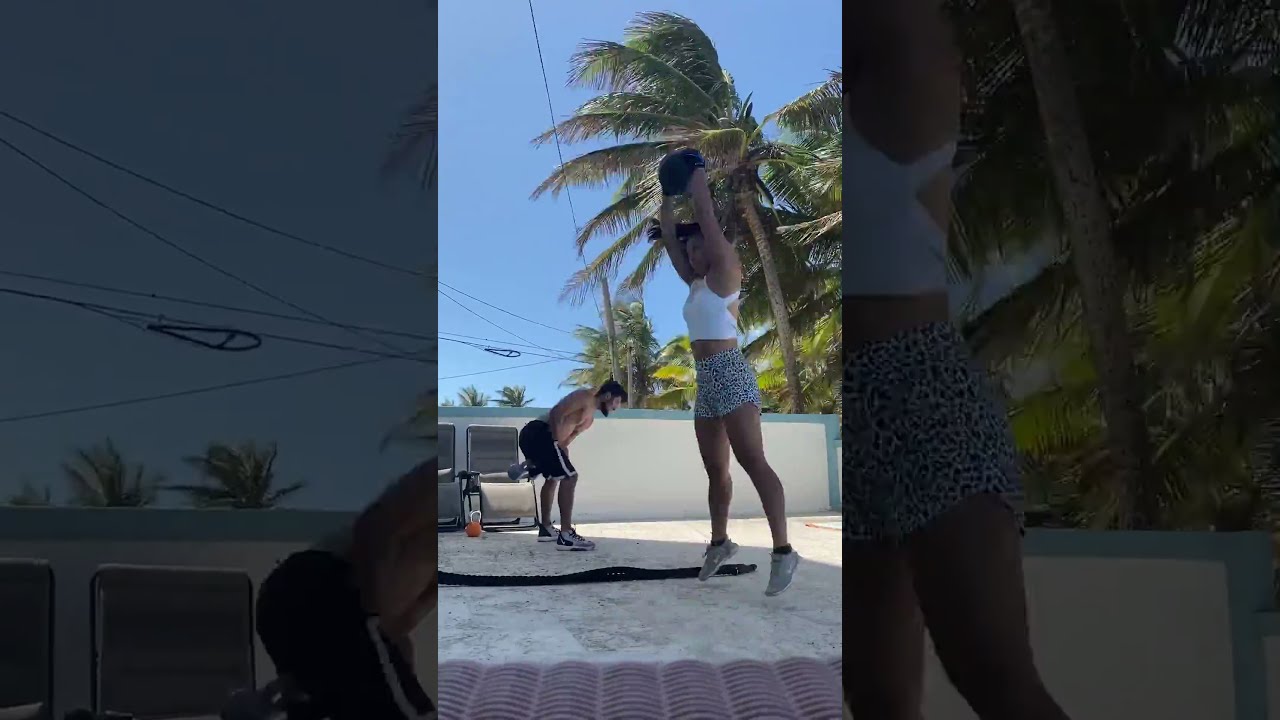In a bright, sunlit backyard area with a waist-high white wall and palm trees against a clear blue sky, two young men engage in a fitness routine. The man in the center, clad in shorts, a white tank top, black ankle socks, and Nike sneakers, holds a basketball while seemingly in a squat position, also sporting workout gloves. Nearby, another young man who is shirtless and wearing black basketball shorts with a white stripe and high-top Nikes points at something off-frame. They are situated on a concrete surface that might be part of a sidewalk, with various fitness equipment such as a disc and a black rope scattered around. In the vicinity, two beach loungers and utility lines are visible. The photo, styled as a vertical cell phone capture, features an artistic touch with a faded, zoomed-in version of the same image as the background, bordered by a pink corrugated scalloped edge.